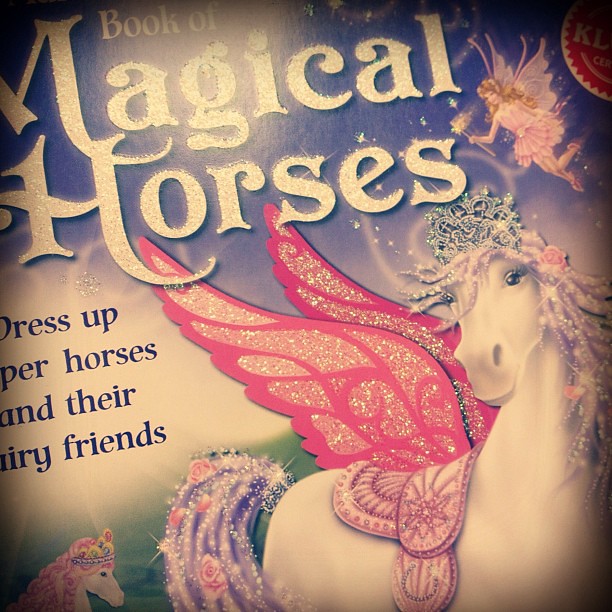The image features a children’s book titled "Book of Magical Horses" against a light blue background. Prominently displayed across the top in bright white letters, the title is accompanied by a depiction of a fairy on the right upper corner. The fairy resembles Tinkerbell, adorned in a pink dress with matching wings, blonde hair, and holding a magic wand.

In the center of the cover, there's a striking white unicorn. This unicorn is decked with a pink and purple glitter saddle, and has pink, purple, and glittering hair. Glittery pink wings extend from its back. Further adorning the unicorn, a diamond tiara rests atop its head, and pink roses are intertwined within both its mane and tail.

Standing behind the unicorn is a regular horse, similar in color but without the magical embellishments. This horse wears a yellow and purple tiara. At the bottom of the cover, a white space in purple letters reads "Dress up horses and their fairy friends," though part of the phrase appears smudged or obscured.

Overall, this enchanting scene is perfectly set for enticing young readers into a magical world of unicorns, horses, and fairies.